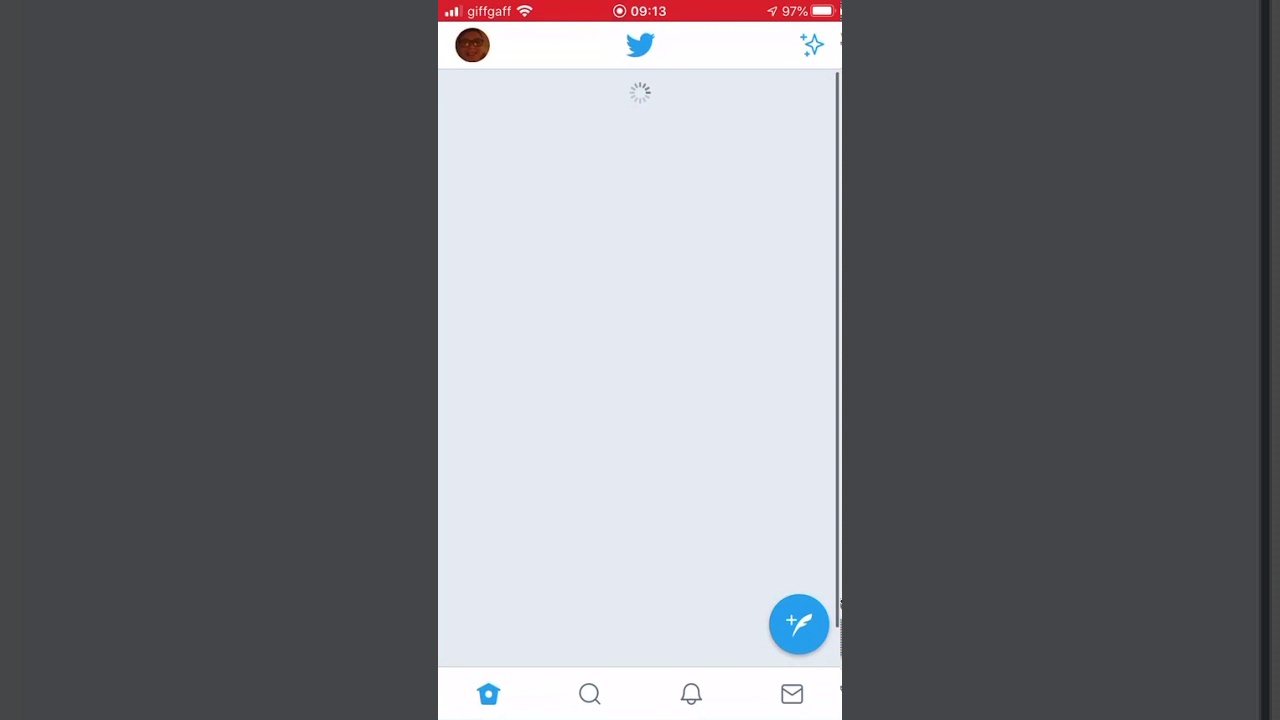A cluttered yet intriguing glimpse into the digital world: The image is a screenshot of a Twitter loading screen viewed through the lens of an art program. The user, identifiable by their glasses reflected on the phone screen, operates their device in Airplane mode, with a 97% battery and uses the GifGaff network. The Twitter app is in a state of limbo; nothing has loaded on the home page, which features the customary home, search, mail, and notification icons at the bottom. Additionally, to the bottom-right, there’s a partially loaded '+' icon with a writing quill in blue. This incomplete interface, coupled with the gray and white blankness, suggests that it’s a screenshot of an already screenshotted image, as evidenced by the two black bars on the sides. This double-layered capture indicates the image was initially taken on the phone and later uploaded into an art-editing program, awaiting further editing.